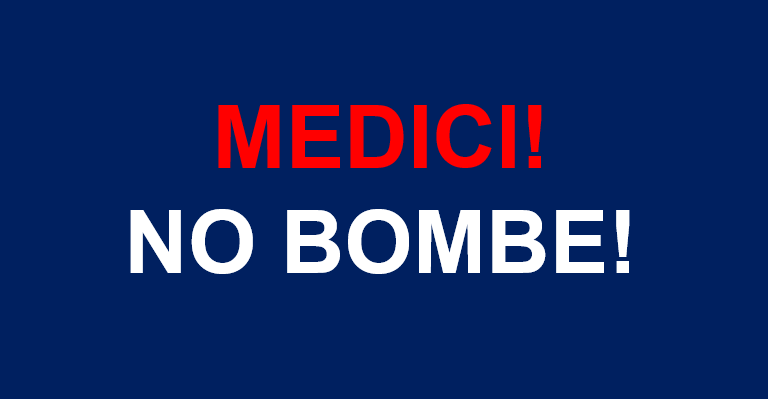The image features a centered rectangular sign set against a solid, dark navy blue background. The sign displays two prominent lines of text in all capital letters, designed to be easily readable due to the high contrast. The first line, "MEDICI!" is rendered in bold red text. The second line, "NO BOMBY!" is in solid white. The two exclamation points further emphasize the message. The words "MEDICI" and "NO BOMBY" are not in English, adding a foreign linguistic element to the design. The overall composition uses a tri-color scheme—blue, red, and white—creating a striking visual effect intended to draw attention and convey an emphatic, clear message.